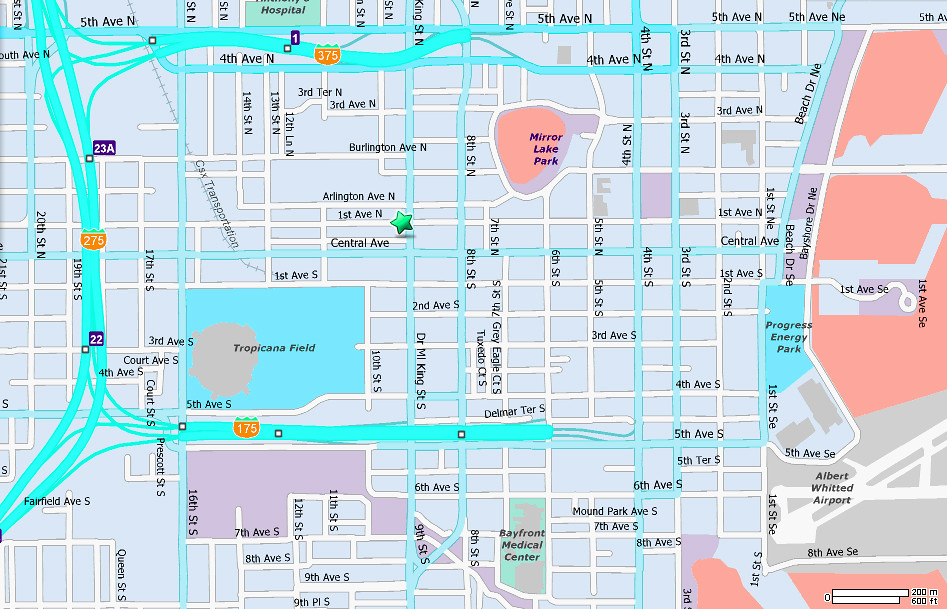The image is a detailed street map featuring a predominantly blue background with an intricate network of blue and green colored highways and roads. To the right, an orange-colored area, possibly an unlabeled park, is depicted. Below this area, Albert Whitted Airport is clearly labeled, complete with a visible runway. Above the airport, Progress Energy Park is identified off of First Street Southeast.

First Avenue Southeast branches from this point, extending both horizontally and vertically in the image. A grid of streets is apparent, including 1st Avenue South, as well as 5th Avenue, 4th Avenue, 3rd Avenue, 1st Avenue, and Central Avenue—all designated with North above Central Avenue.

Mirror Lake Park is prominently marked towards the top center of the map. On the left side, near the bottom, Tropicana Field stands out in blue; the surrounding streets either end at or border this large venue. Additionally, a freeway marked as I-275 runs through the map, further delineating the area's infrastructure.